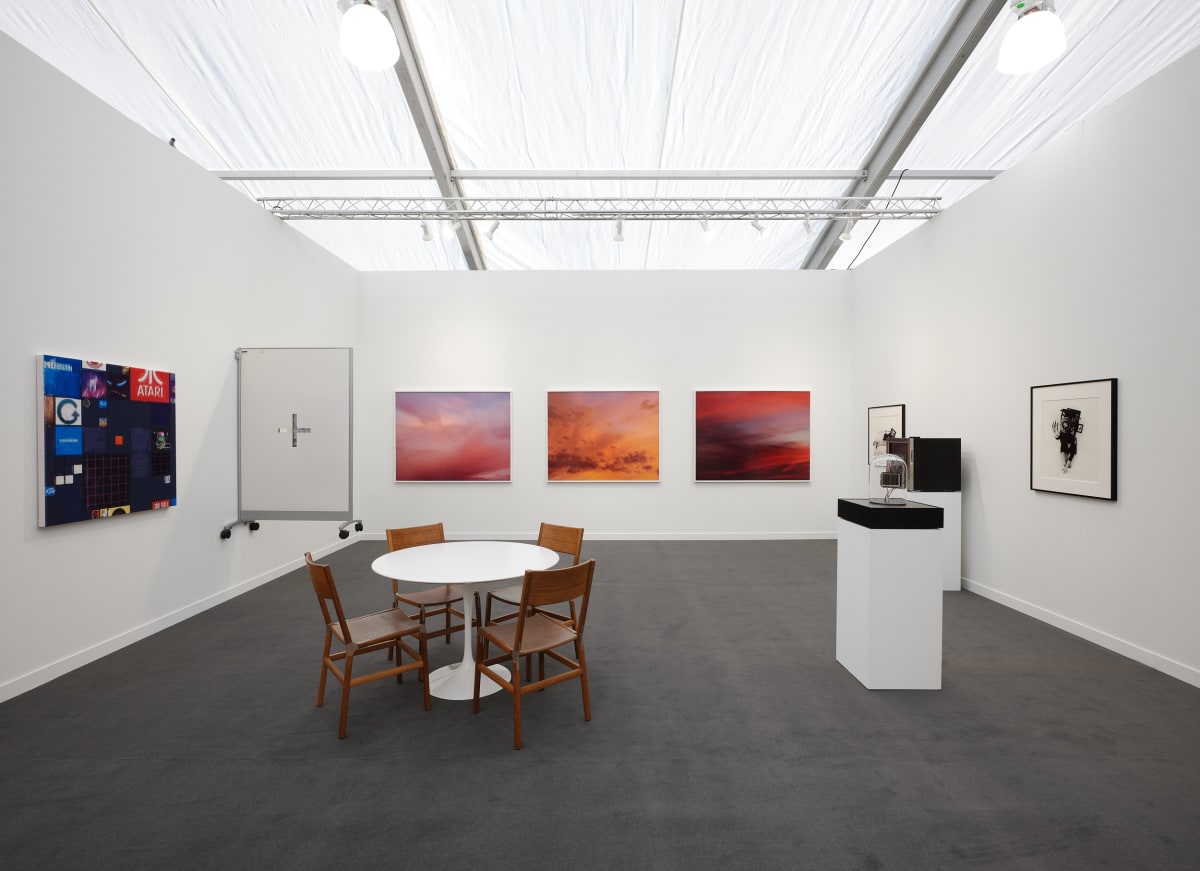The image is an indoor, artificially-lit room with a white, textured ceiling intersected by metallic girders. Overhead lights are visible, casting light onto the scene. The room is encased by three white walls adorned with various artworks. The left wall features a colorful display including logos such as Atari and Google, possibly on a monitor screen. The back wall displays three vibrant, colorful swatches resembling sunset skies. The right wall is decorated with two black-and-white photographs.

In the center-right part of the room, slightly detached from the walls, there is a white sink with a black countertop and a faucet. The floor is gray, and a white, round table with four wooden chairs is positioned centrally. The overall setting suggests an exhibition or gallery space, as there are no people present, and the artworks are prominently displayed for viewing.